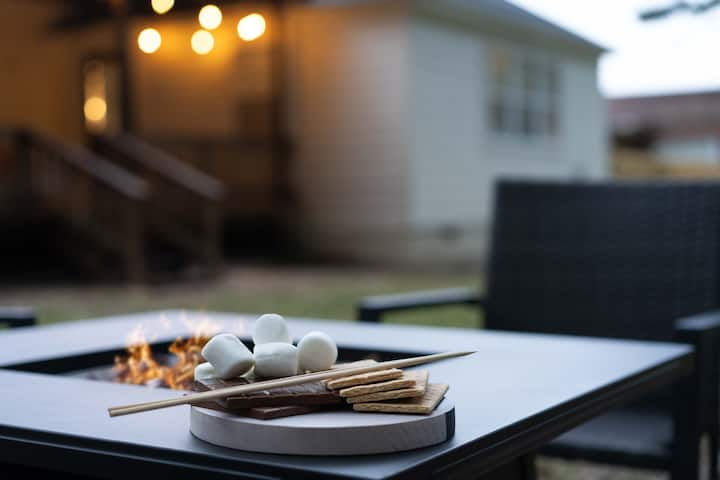This outdoor backyard photograph captures a black, almost square table featuring a central fire pit emitting flames. On the front corner of the table sits a small, round, white ceramic plate adorned with ingredients for making s'mores: marshmallows, Hershey's chocolate bars, and graham crackers, with wooden chopsticks laid across them. A slightly blurred black chair is positioned behind the table. The background reveals a blurred image of a white house with a staircase leading to the front door, adorned with multiple porch lights on the ceiling. The ground area surrounding the house is blanketed in green grass, and the overcast sky adds a grey tint to the scene.